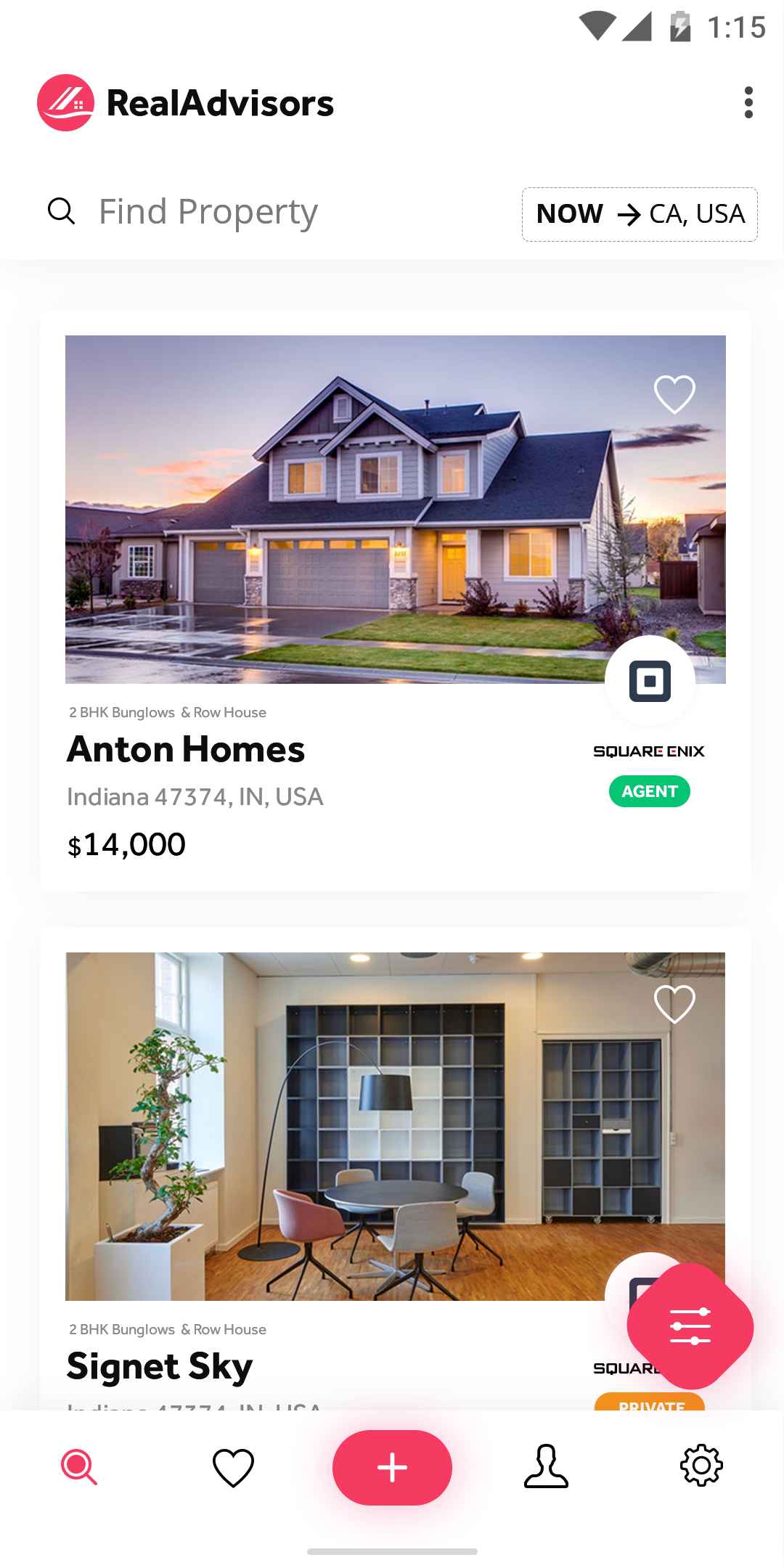The image displays a home advertisement viewed on a mobile phone. The screen shows the typical icons for Wi-Fi and battery status, along with the time which reads 1:15. 

At the top in bold, small, black text, it reads "Real Advisors" next to a red icon with a white house silhouette. Below this, there's a search bar with an icon resembling a magnifying glass, labeled "Find Property Now". The location is marked as "CA, USA".

The advertisement features an image of a property described as a "2BHK bungalow and row house", listed under "Anton Holmes". The address provided is "Indiana, 47374, IN, USA". Further down, there is a partially obscured line that mentions something about an agent.

At the bottom of the advertisement, there’s another image showing an indoor room resembling a conference room. This room contains a table with four chairs arranged around it, and several empty shelves. The room has a hardwood floor and includes a small planter with a tree that has green leaves growing in a slightly crooked fashion.